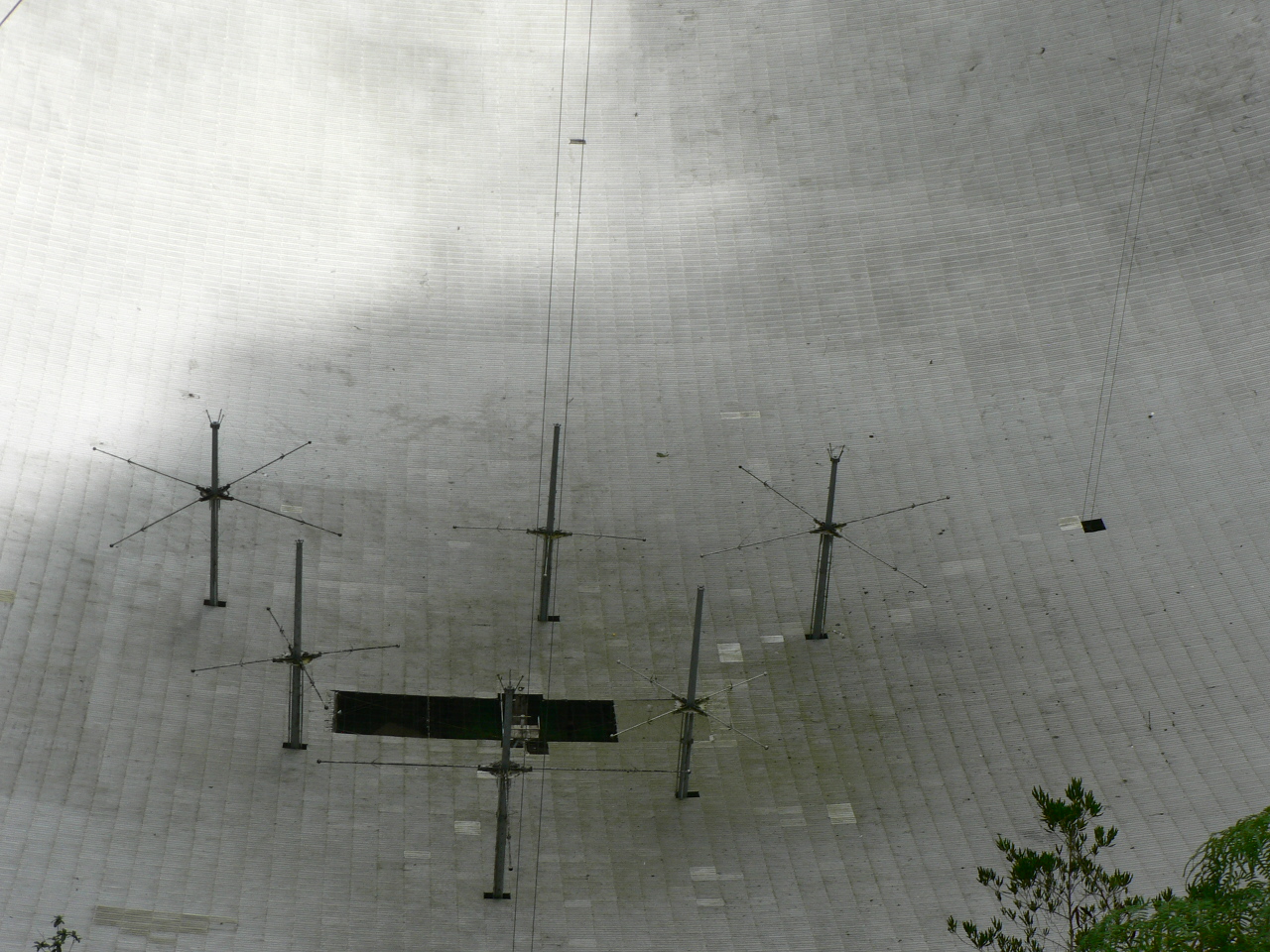This overhead color photograph captures a complex arrangement that appears to be a large satellite dish or a set of interconnected antennae rather than a wind turbine farm. The focal point of the image consists of six small metallic micro-antennae arranged in a triangular pattern, from smallest at the bottom to largest at the top, set on a structure that features more antenna poles projecting from its sides. The metallic objects create a cross-sectional alignment in the central area. 

The backdrop involves long, large, interconnected white panels extending in multiple directions, adding to the complexity and the sense of scale of the satellite apparatus. The tall central wire and the X-shaped formation of metal stands dominate the scene, hinting at this being a sophisticated signal or attention-boosting device. 

There is a noticeable reflective or misty area in the top left corner, giving an overcast and gray ambiance, as if clouds or steam are present. The overall color scheme is predominantly silver, gray, and white, with patches of green moss or growth in the center, suggesting some weathering or biological interaction. The presence of green tree branches entering the bottom right and potentially bottom left corners confirms the outdoor setting. The ground appears white, possibly composed of stones or perhaps dead grass, adding to the scene's enigmatic and intricate nature.